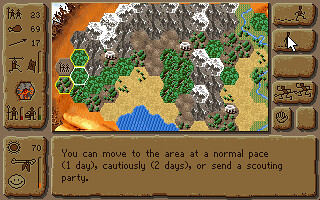The screenshot from the video game presents a detailed, cartoonish aerial view of a prehistoric map in the center, featuring brown-colored mountains with gray tops, possibly to signify snow. On the left side of the map, yellow-outlined hexagons filled with green suggest areas with trees. At the bottom, a blue river with lines passes through, zigzagging across the screen, depicting water. Surrounding the map are various interface elements: brown-colored buttons on both sides and additional buttons in the upper right corner with different icons such as a person walking, two people running, a hand, and a blank button.

On the left side of the screen, numbers are placed beside various primitive symbols and etchings: the numbers 23, 69, and 17 appear adjacent to depictions of people and objects like a turkey leg. Below these, an area showing a sun with the number 70 next to it, and a bone wrapped with red fabric sits above a power bar barely filled with orange. The bottom left corner hosts a circle with a smiley face.

A dark brown rectangle stretches across the bottom, containing text options for movement: "move to the area at normal pace, cautiously, or send a scouting party." This detailed layout conveys the game’s setting, depicting tribal life and exploration of the natural landscape.